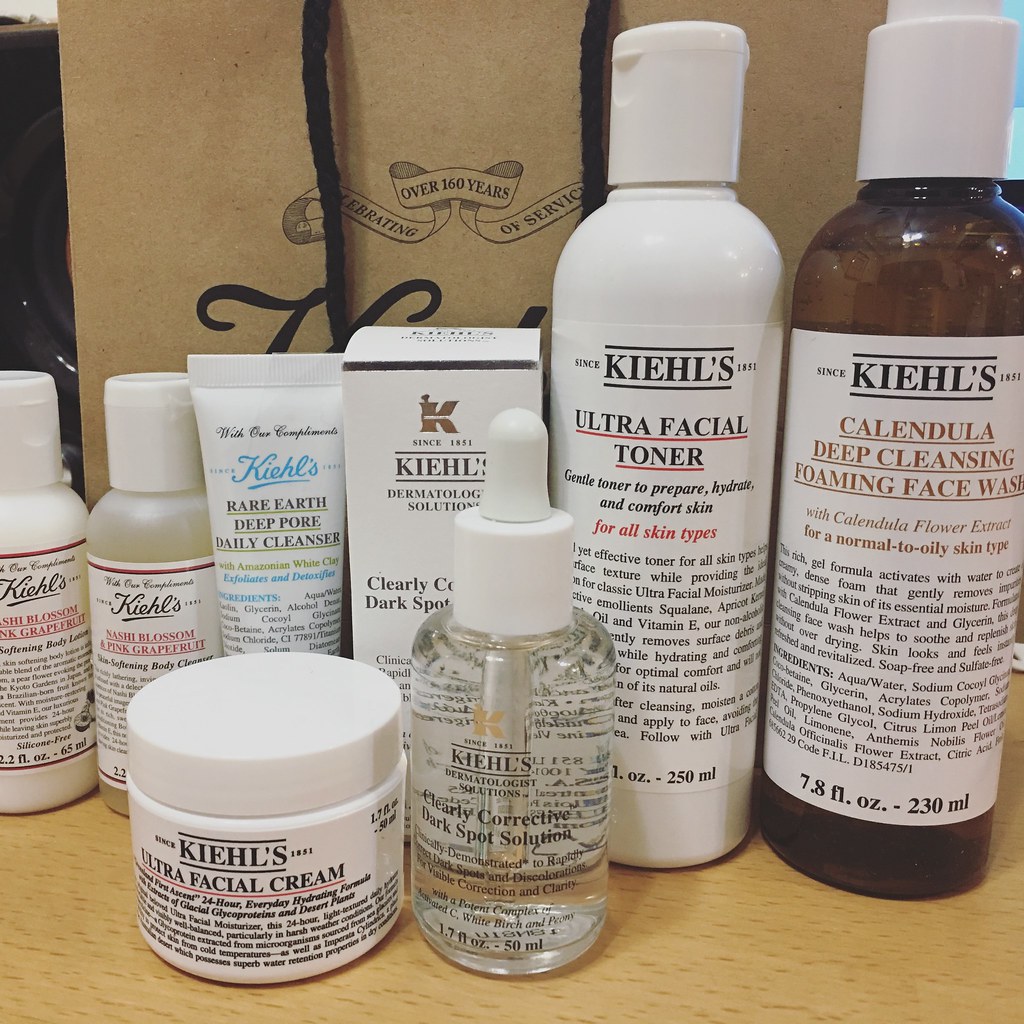A collection of Kiehl's skincare products beautifully arranged, showcasing an array of face care essentials. The assortment includes cleansers, toners, moisturizers, and serums, each in their distinctive packaging adorned with the brand's iconic labeling. The products, varying in sizes and shades, are meticulously placed against a clean, neutral background, highlighting the brand name "Kiehl's" with its signature apostrophe and elegant typography. The composition emphasizes the diversity and premium quality of Kiehl's offerings, catering to a comprehensive skincare routine.